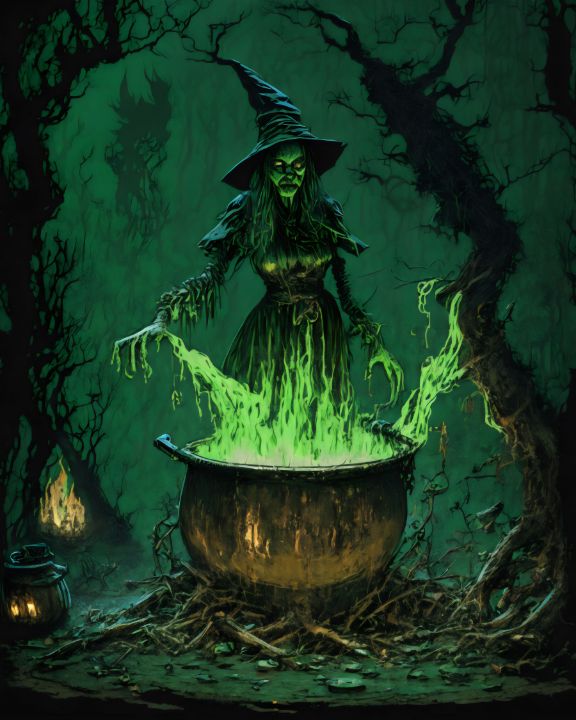This haunting painting depicts a sinister witch standing over a large, fiery copper cauldron with green flames and smoke rising out. The eerie background features a deep, foggy green forest filled with gnarly, leafless black trees that contribute to the nighttime, spooky atmosphere. In the distance, a small fire flickers by one of the trees, adding to the unsettling scene. The witch, clad in a long black dress with a very tall pointy hat, has bony skeleton-like hands and a ghastly green face with hollow eyes, and her stringy hair drapes down on both sides. She peers down at the fire with a malevolent expression, embodying the quintessential evil witch. The gnarled sticks beneath the cauldron and small pot on the ground enhance the eerie forest setting while tiny lanterns dot the scene, casting an additional ominous glow.